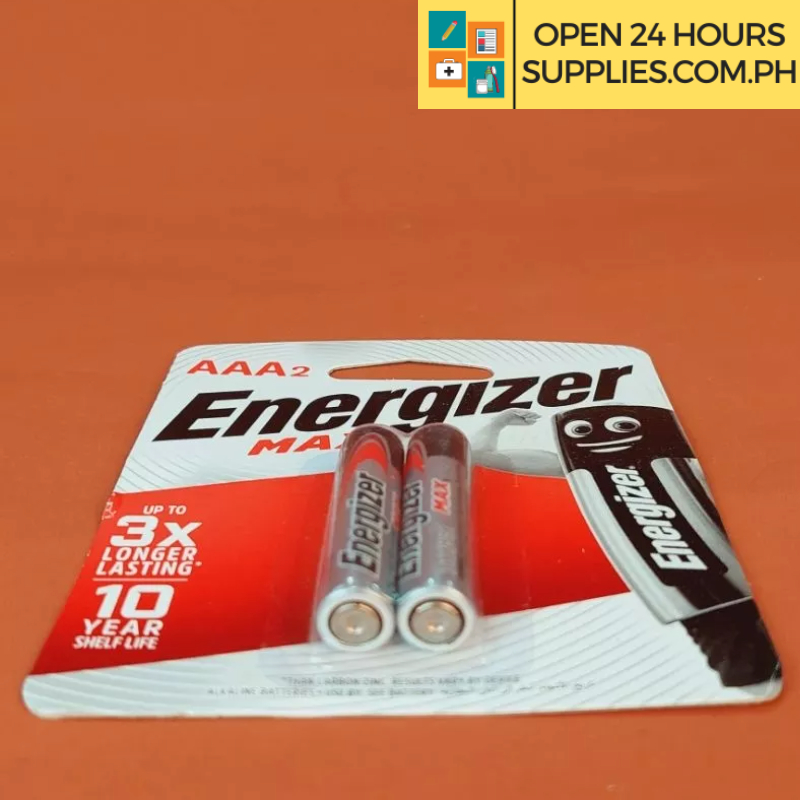In this detailed image, we observe a package of AAA batteries prominently displayed. The background features a brownish-orange hue. Positioned at the top right corner, there is text that reads "open 24 hours supplies.com.ph" in black font against a white rectangular backdrop. Adjacent to this text on the left, there's a vertical black line followed by four small squares—two orange and two blue—each containing distinct icons.

The package is viewed from the front, lying flat so the top is visible. The bottom section of the packaging is white with thin lines overlaying it. The two batteries housed within are primarily gray with a touch of red, and their tops are black, each branded with the word "Energizer" in black text.

On the left side of the packaging, white text proclaims "up to 3X longer lasting" and "10 years shelf life." To the right, there is an Energizer battery logo depicted as a character flexing its arm, colored in black and light gray. Across the top of the package, red text indicates "AAA2," confirming the type of batteries enclosed.